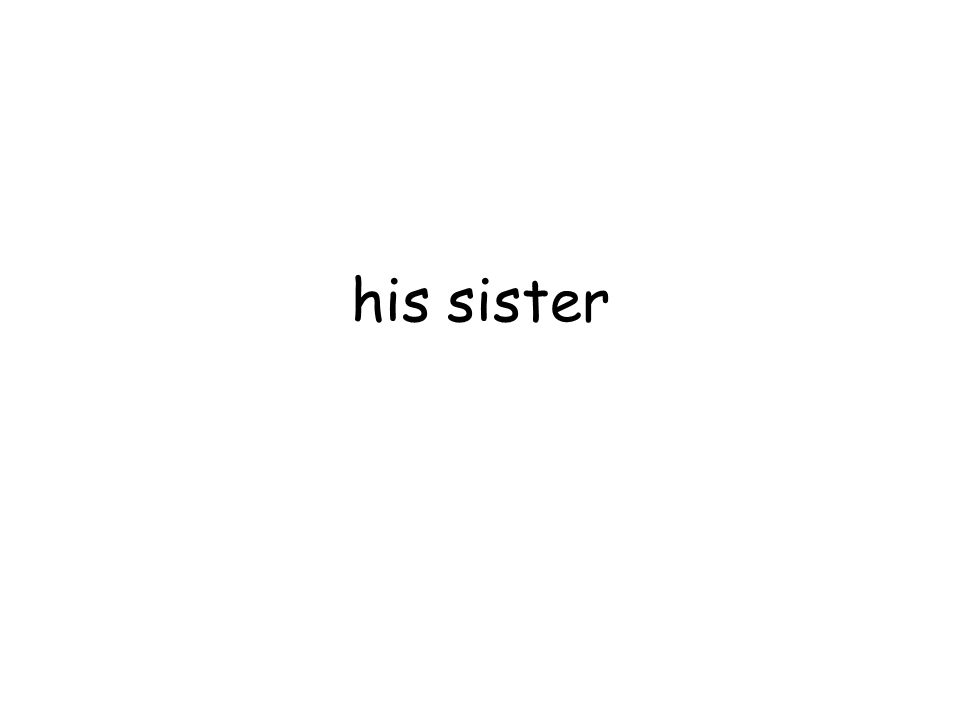The image features a stark, white background devoid of any borders or additional elements. At the center, two lowercase words, "his sister," are displayed in a thin, black font that is uniform and slightly rounded, indicating it was not hand-written. The letters are consistent, with each "s" appearing identical to the others, further emphasizing the mechanical precision. The simplicity of the composition draws focus squarely on the text, making it the main and only subject of the image.